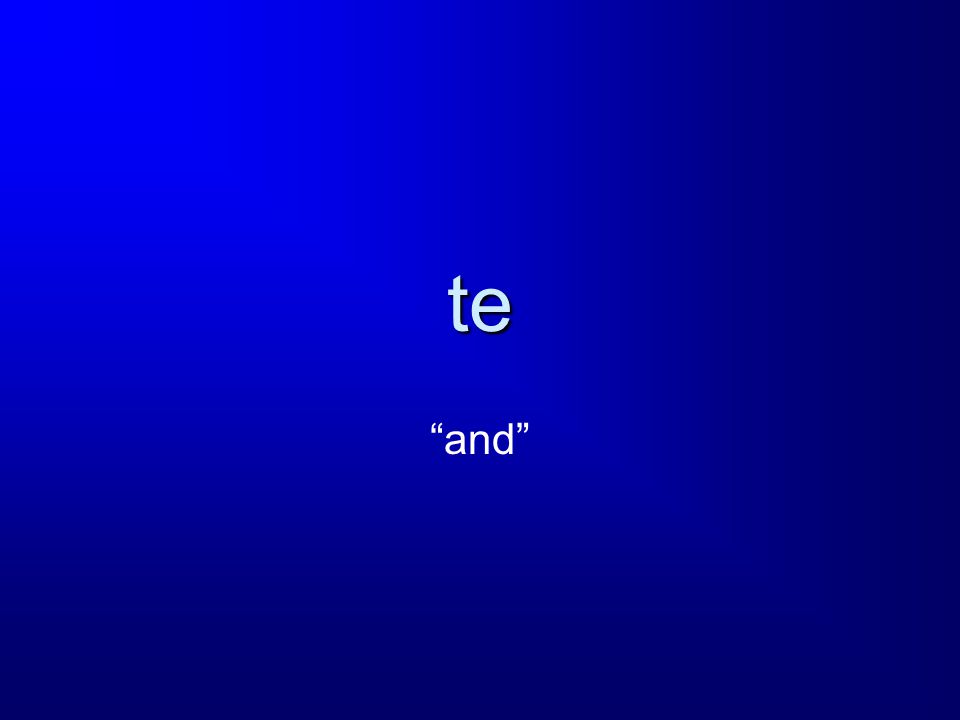The image is a square with varying shades of blue: darker blue on the bottom and top right, and a brighter blue on the top upper part. The image's background transitions from dark to light shades of blue, adding depth to the otherwise simple design. At the center of this blue square, there are two white, lowercase words which are horizontally aligned. The top word is "te," and just below it is the word "and" in quotation marks. The overall style suggests the image is related to language or translation, possibly illustrating that "te" means "and" in another language. The clean, minimalist design and subtle color gradients give it a modern, website-like appearance.